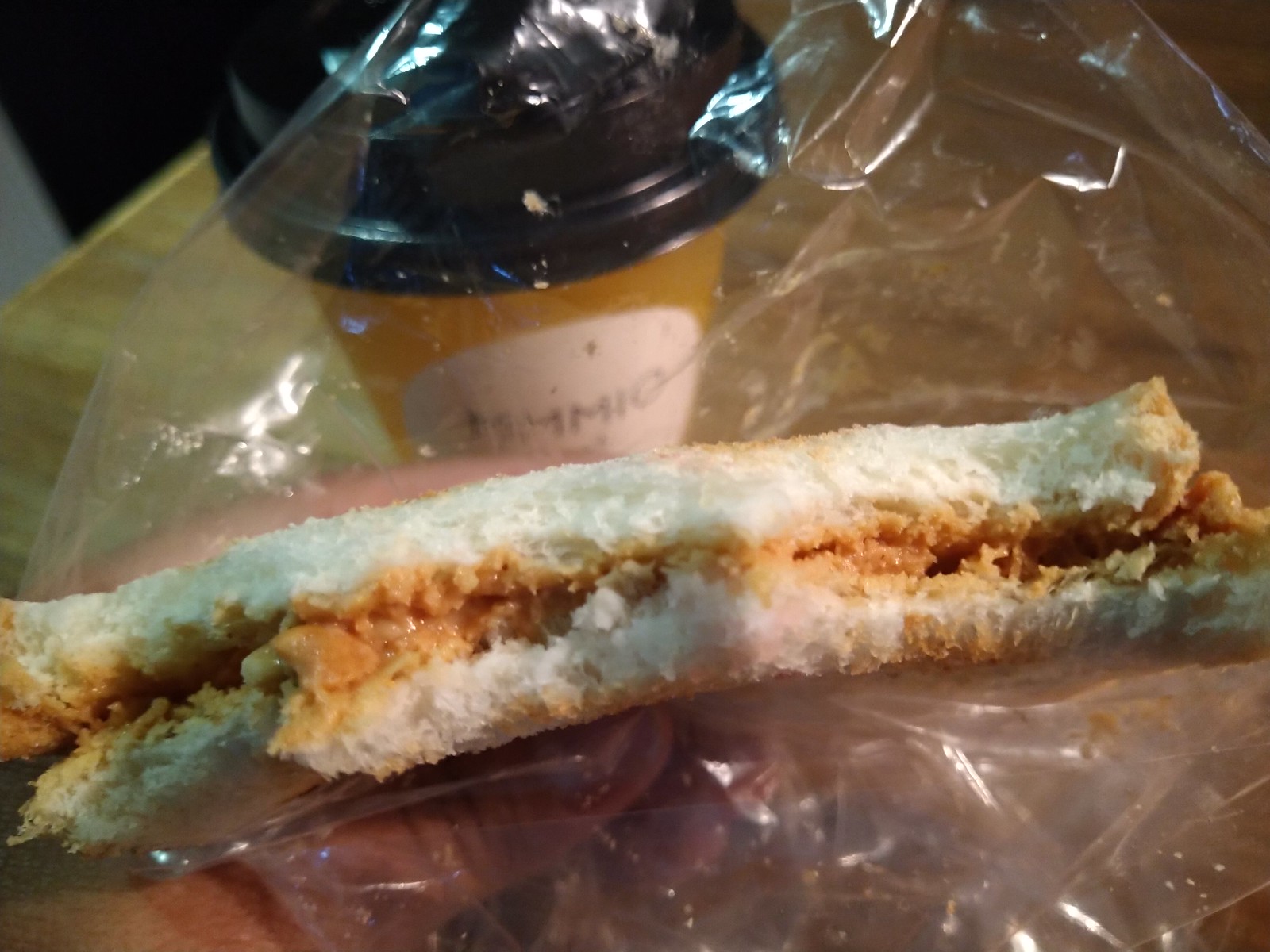The close-up photograph captures a mostly eaten peanut butter sandwich, partially encased in clear, reflective plastic wrap. The sandwich is composed of two slices of white bread with light brown crusts, visibly showing teeth marks from being chewed across from left to right. A light-skinned person's thumb and index finger are seen partially underneath the sandwich, holding it delicately. Behind this, on a light brown wood table, sits a to-go coffee cup with a black lid and tan sleeve. The cup features a large white circle with black text that reads "MMIO," though the first few letters are obscured by the plastic around the sandwich. The overall scene is an intimate snapshot of a mid-snack moment.